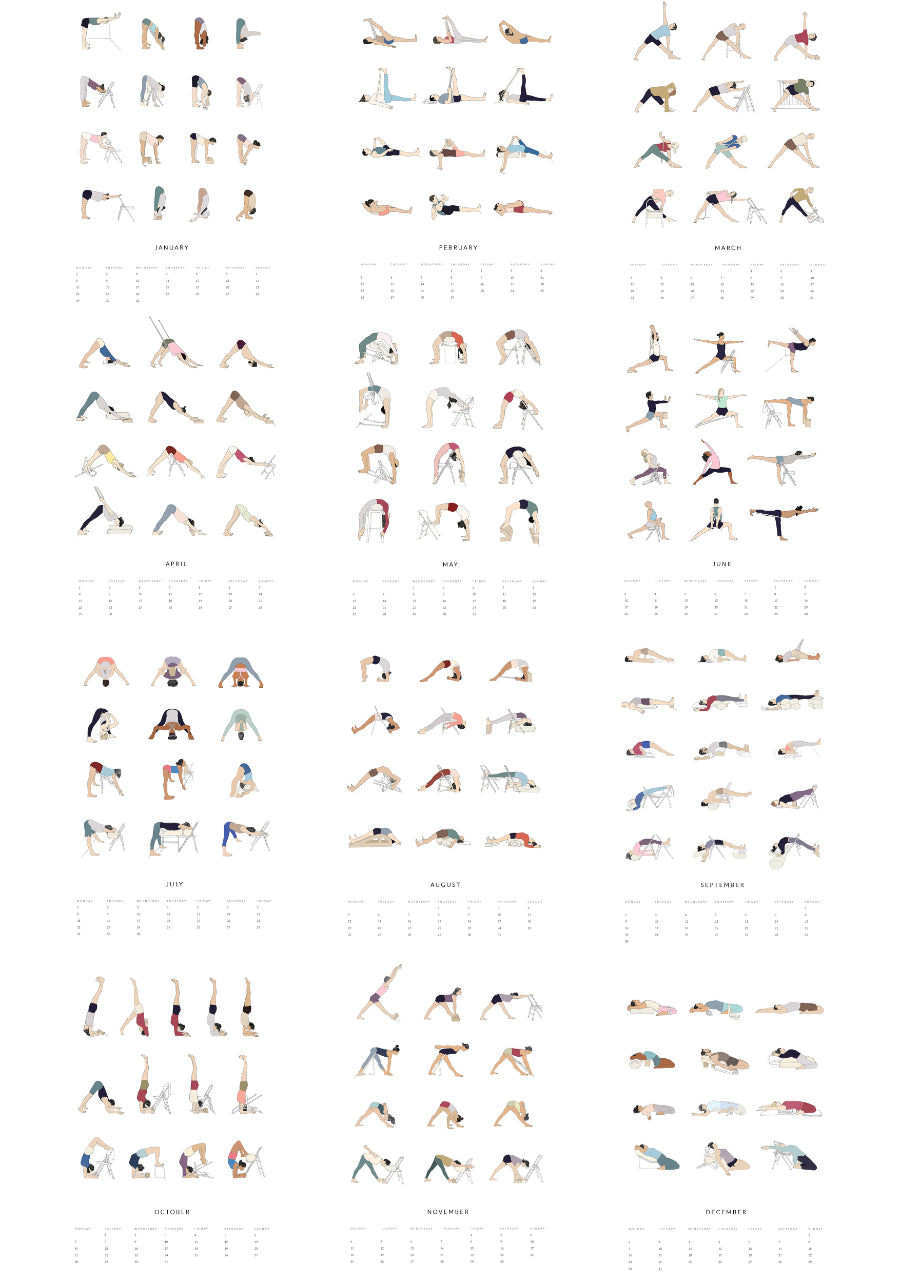This is a detailed color illustration of a calendar presented in a grid format with 12 squares, each corresponding to a month from January to December. Each square contains a depiction of people performing various exercise and yoga poses, arranged in four rows of four illustrations. The calendar is laid out in three rows with four months on each row, making a clear, organized visual sequence.

- **January** shows individuals bending over, touching their toes.
- **February** features people lying down with their legs raised in the air.
- **March** depicts figures bending to the right with one arm up and their legs spread.
- **April** shows participants in a downward dog yoga pose.
- **May** displays individuals performing back bends.
- **June** showcases a variety of yoga poses, some of which appear to defy gravity, giving a “flying” impression.
- **July** illustrates people bending forward with their legs spread and arms around the back of their legs.
- **August** has individuals on their backs with heads to the ground and bodies bent upwards.
- **September** features people lying on their backs with their midsections lifted into the air.
- **October** depicts handstands.
- **November** shows individuals leaning forward, touching their feet or reaching towards the ground.
- **December** highlights people on their knees, bending backwards with their feet behind them.

Underneath each exercise illustration is a faint and small text indicating the respective dates and days of the week for each month, although the text is difficult to read. The overall layout suggests this calendar could be used in an exercise or yoga class setting to depict different poses associated with each month.